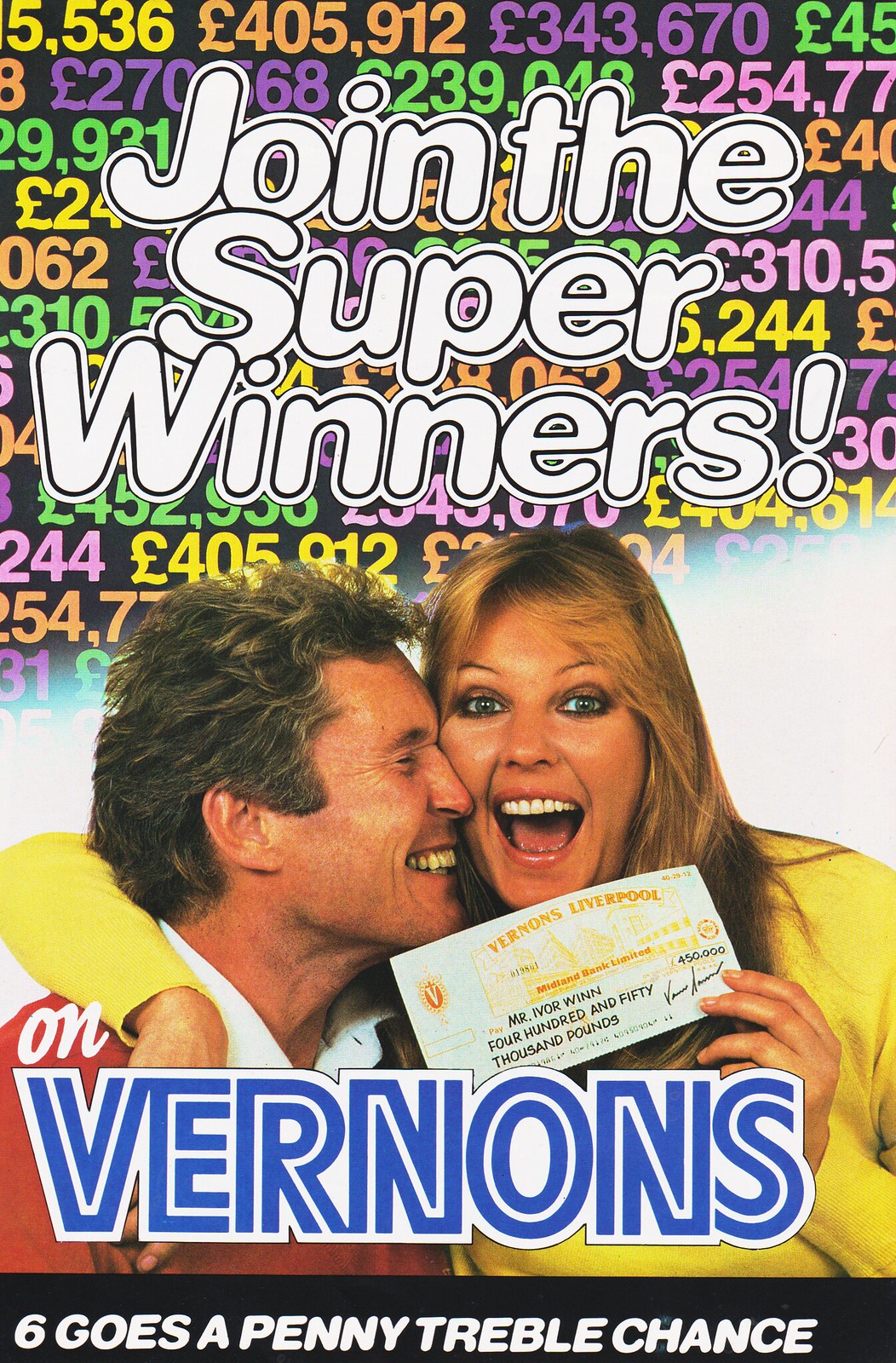The image is an advertisement for a lottery or gambling promotion by Vernons. At the top, bold white bubble letters on a black background with colorful numbers read, "Join the Super Winners." Below this headline, a jubilant couple is featured. The man, wearing a red shirt with a white collar, stands to the left, facing the woman. His profile is visible, showcasing his broad, toothy smile. The woman, with blonde hair and a yellow blouse, stands to the right, facing the camera with an open-mouthed, ecstatic expression. She is holding up a large check that appears to be from Vernons, Liverpool, issued by Midland Bank Limited, showing a prize amount of £450,050. Just below their chins, text in a smaller font reads "on Vernon's." At the bottom of the advertisement, a black box contains the phrase, "six goes a penny, treble chance." The overall scene captures the excitement and joy of winning, with an emphasis on the substantial prize amount and the celebratory mood of the winners.